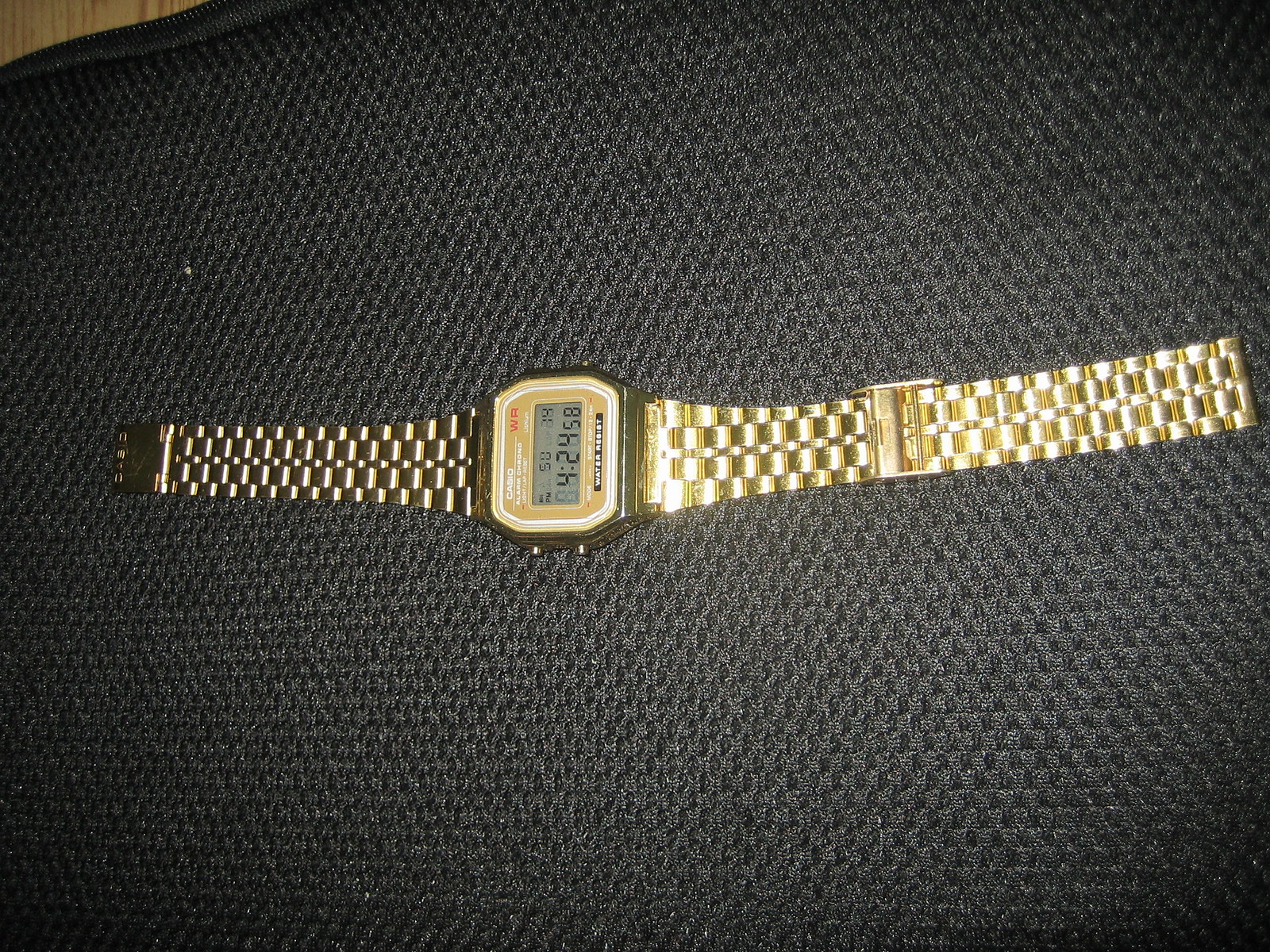This photograph features a meticulously designed digital watch set against a sophisticated black background, embellished with a subtle pattern of raised, darker black squares. The watch lies flat, oriented horizontally across the image. Its face is a striking square design, framed with gleaming gold metal. Inside this frame, a delicate white line outlines the watch face, which is filled with a rich, deep tan hue. On the upper left side of the face, white text provides a crisp contrast. Central to the watch face is a digital display, characterized by a muted gray-green background. The watch band is composed of interlinked gold metal segments, accentuated by yellow pins, adding to the overall luxurious appearance.